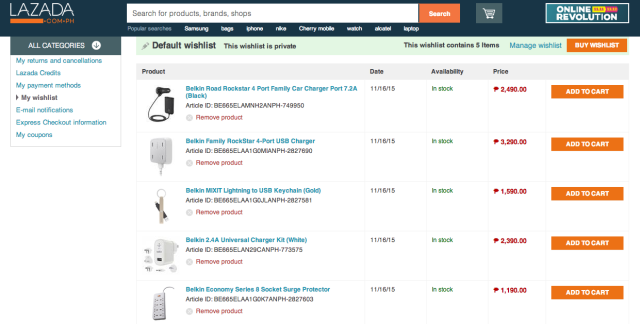The image showcases a busy and colorful webpage layout. At the very top, there is a blue rectangle featuring the word "Lasda" in white text. Directly beneath it, there is an orange rectangle that contains no visible text. Below this, a white rectangle contains some text, and next to it is another orange rectangle, likely indicating a "search" function.

Further down, white text is visible under the white rectangle. Adjacent to this, there is a light blue-green rectangle containing an indistinct picture. Next, there is another rectangle outlined in white transitioning from light blue-green to darker blue, with the words "Online Revolution." This section also features two small rectangles in orange and red, each containing text.

On the left-hand side, a green rectangle is labeled "All Categories," beside a white circle with a symbol inside. Below this, there are blue words, except for one in black in the middle. Following this, a light green rectangle includes the words "Default" and "Wishlist," along with more black text, blue text, and an orange rectangle with additional words.

A gray rectangle on the page displays headers such as "Product," "Date," "Availability," and "Price." Below this, there are five repeated sections, each containing:
1. An item picture.
2. A description in blue and black text.
3. Some text in red.
4. A date.
5. Text in green and additional red text.
6. An orange rectangle labeled "Add to Cart."

These sections consistently provide a product image, description, date, availability status, and an option to add the item to the cart, ensuring a structured and detailed presentation of products for online shoppers.